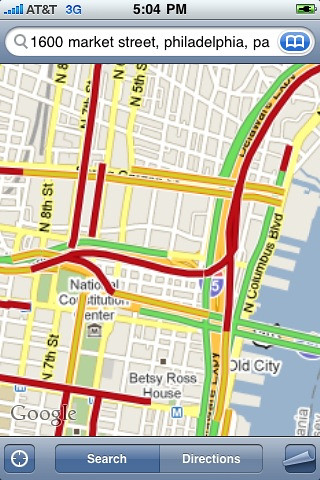The image features an AT&T phone running on a 3G network, displaying a map centered on 1600 Market Street, Philadelphia, Pennsylvania. The map, viewed at approximately 5:04 - 5:05 p.m., showcases various roadways and pathways. The streets are depicted in different colors—red, yellow, green, and orange—likely indicating traffic conditions or route options. Landmarks such as the Betsy Ross House are marked on the map, though specific street names and the exact location of 1600 Market Street are not prominently labeled, contributing to some ambiguity.